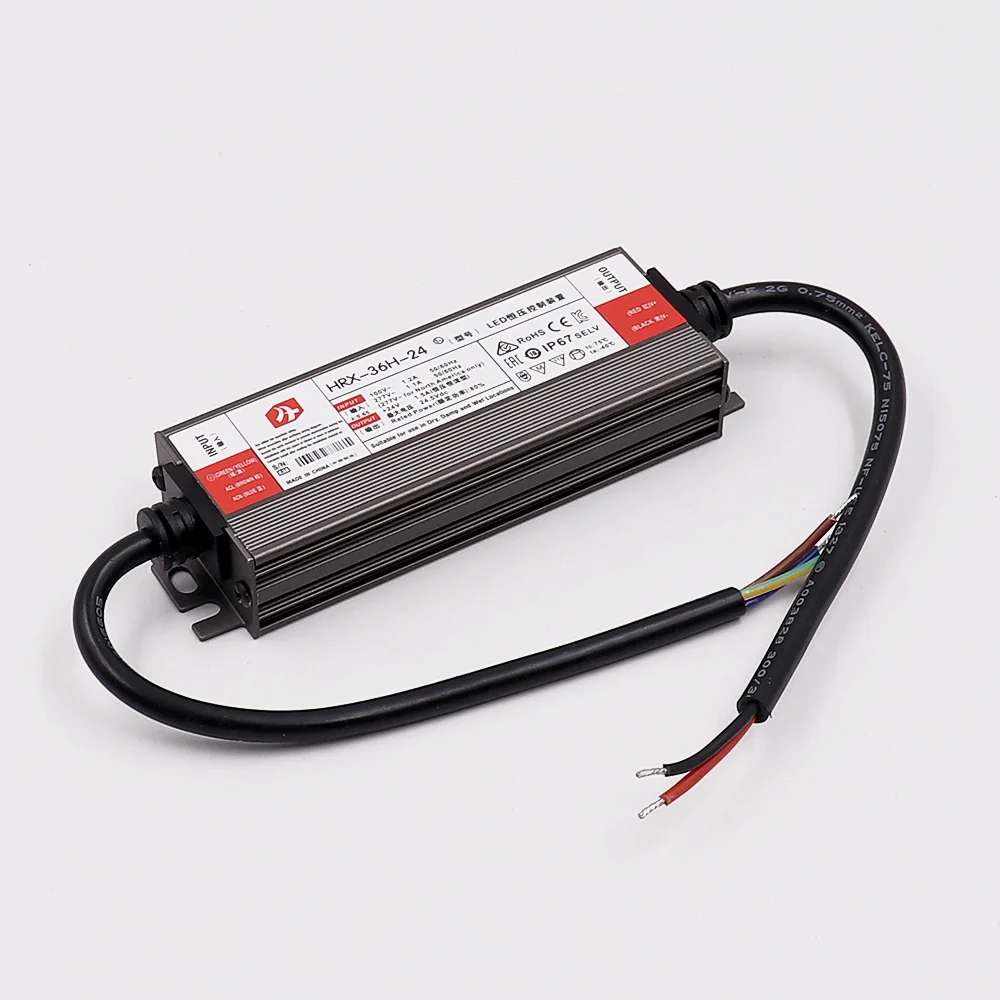This is a square color photograph of an LED transformer, possibly a power supply or a low voltage meter, set against a light gray background. The subject is a black rectangular electronic device, positioned diagonally with its short sides facing the bottom left and top right corners of the image. Two thick black cables extend from either side of the rectangle, curving around to the front. The cables' sheaths have been partially removed to reveal the colored wires inside; on the visible front side, there are red and black wires, while the opposite side showcases additional wires including red, white, and at least one more color. A label spans the top of the black case, featuring the text "HRX-36H-24" along with characters that appear to be in Japanese or Chinese, providing usage instructions and statistical information. The image, rendered in a style of photographic representationalism and realism, focuses on the detailed presentation of the electronic equipment.